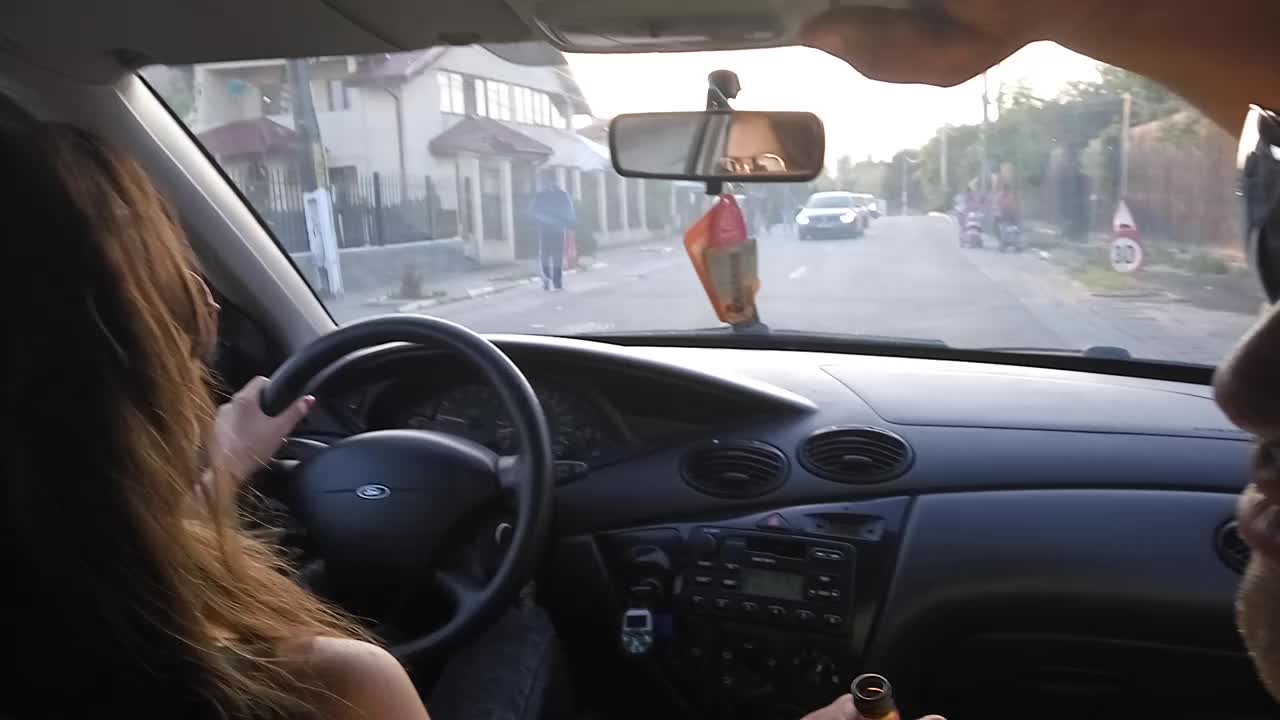In this photograph, captured from inside a car, a woman with long brownish-blonde hair is driving, her hand securely placed on the steering wheel of a Ford vehicle. The car's interior is sleek in black. Seated beside her is a man, engaged in conversation, and holding a bottle in his hand. The car's rearview mirror reflects part of the scene, adorned with something pink hanging from it. Ahead, a building appears on the left with a pedestrian walking along the sidewalk, while cars approach from the opposite direction. To the right, a fence lines the road, and a speed limit sign marked '30' in a red and white circle is visible. Power poles stand tall in the distance as the woman drives along the road.